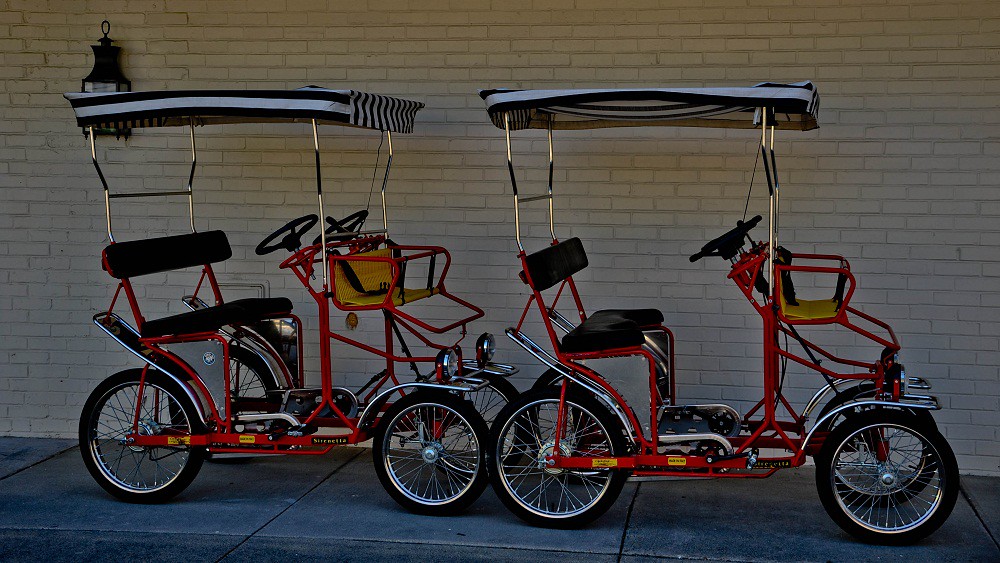The image depicts two fascinating, red-framed quadricycles parked in a row, one directly behind the other, set against a pale ivory brick wall on a large, dark gray tiled surface. These vehicles, resembling a mechanical blend between two bicycles and an open golf cart, are designed with four wheels each, featuring black tires and silver spokes. Each quadricycle includes two black seats and two individual steering wheels, under a blue and white striped canopy supported by a metal frame. The front of the vehicles is equipped with yellow baskets, which may serve as child seats complete with seat belts and leg straps. Despite being dimly lit, potentially due to an overcast sky, the photo is sharply focused and well-framed, capturing the unique design and recreational essence of these multi-passenger pedal-powered buggies, typically found at fun fairs or in parks.